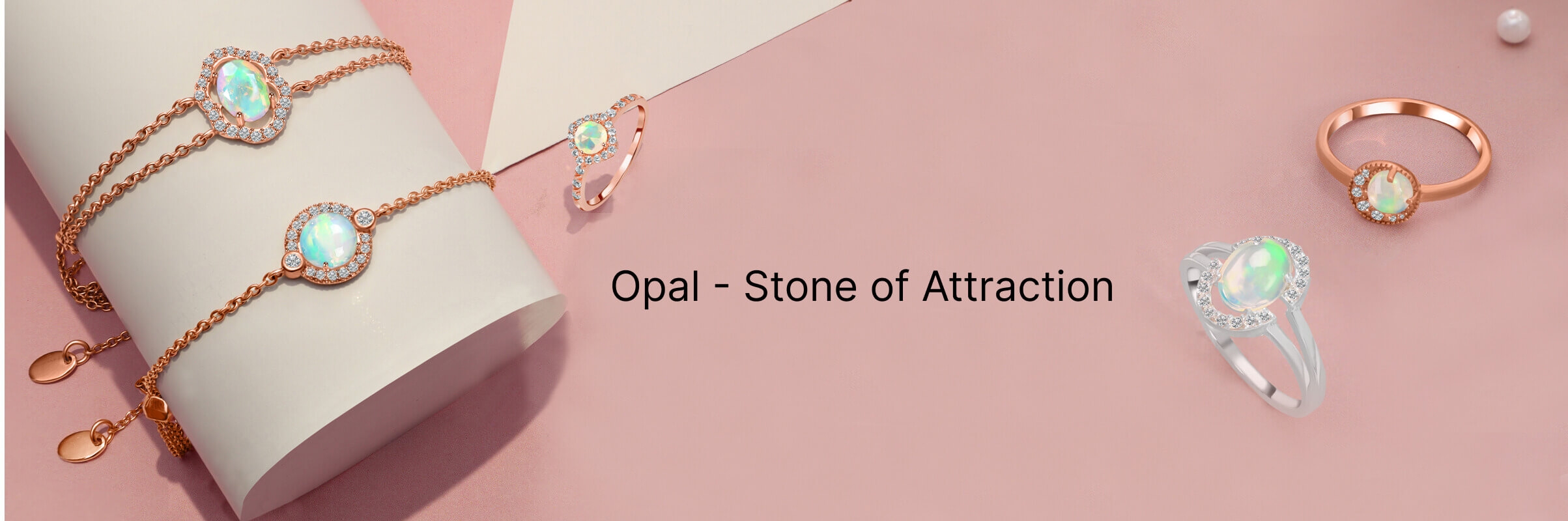Set against a vibrant pink background, this image showcases an exquisite array of jewelry highlighted by the central text, "opal - stone of attraction" in bold black letters. At the upper right corner, a lustrous white pearl gleams, closely accompanied by a stunning gold ring adorned with a central diamond encircled partially by smaller diamonds. Below and slightly to the left of the gold ring, a silver ring featuring an opalescent center displays a beautiful white and greenish glow. 

To the left of this silver ring, a white display piece holds two elegant gold bracelets. The lower bracelet, characterized by a single strand chain, features a central gem that exhibits a white and turquoise radiance, likely an opal, surrounded by a circle of tiny diamonds. Above it, an oval-shaped bracelet with a double strand design mirrors the lower one with its glowing opal centerpiece, similarly adorned with surrounding diamonds. The entire collection exudes an air of refined elegance, underscored by the opals' mesmerizing allure.